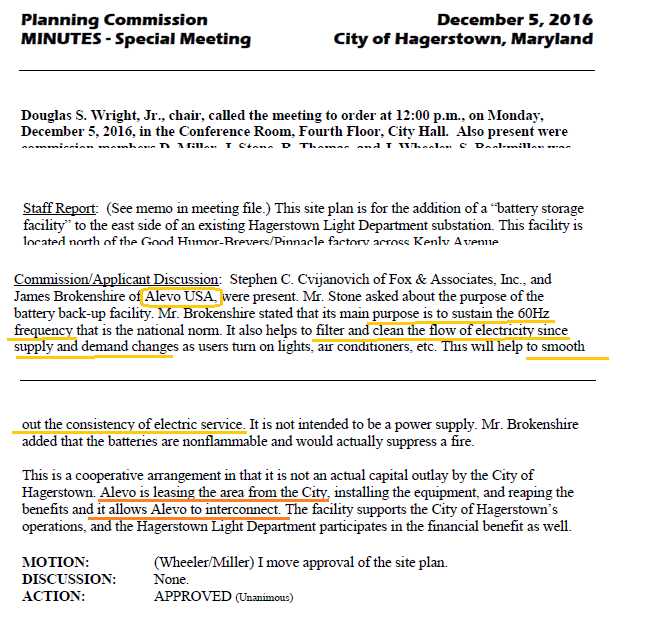These are the minutes from a Planning Commission Special Meeting held on December 5, 2016, for the City of Hagerstown, Maryland. The minutes document the proceedings presided over by Douglas S. Wright, Jr., Chair, who called the meeting to order at 12 p.m. in the conference room on the fourth floor of City Hall. The meeting focused on the approval of a site plan for the addition of a battery storage facility to the east side of the existing Hagerstown Light Department substation. This facility is planned to be located north of the Good Humor Breyers Pinnacle factory, across Kenley Avenue. Steven C. Sijanovich of Fox and Associates, Inc., and James Brokenshire of Alevo, USA, were present to discuss the project, which aims to sustain the 60-hertz frequency that is the national norm and to filter and clean the flow of electricity. The facility will help smooth out the consistency of electric service rather than serve as a power supply. Brokenshire highlighted that the batteries are non-flammable and would suppress a fire, emphasizing the safety and cooperative nature of the project. The minutes record the motion for approval of the site plan, noting "I move approval of the site plan," with no further discussion, and the action was approved unanimously. The meeting adjourned at 12 p.m.